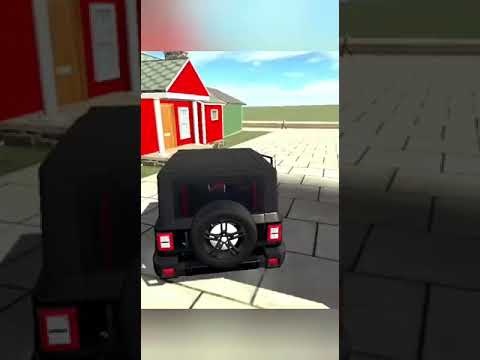A screenshot from a video game animation depicts a black Jeep, with a cloth top and a spare tire on the back featuring a white circle in the middle. The Jeep's rear showcases taillights that include two white squares on each, and additional red lights located on the corners of the black bumper. The vehicle is turning onto a pathway made of white square tiles secured by dark grout. Directly in front of the Jeep is a prominent red house with gray shingles on the roof, a brown door, and a white window. To the side of the red house is a green building with a sharply angled roof. In the distance, a person appears to be moving across the pathway where it intersects in a T, under a sky that is mostly blue with some surrounding clouds. The scene reflects a simplistic, cartoon-like aesthetic reminiscent of games such as Fortnite, with no trees in sight, just green land stretching out under the blue sky.